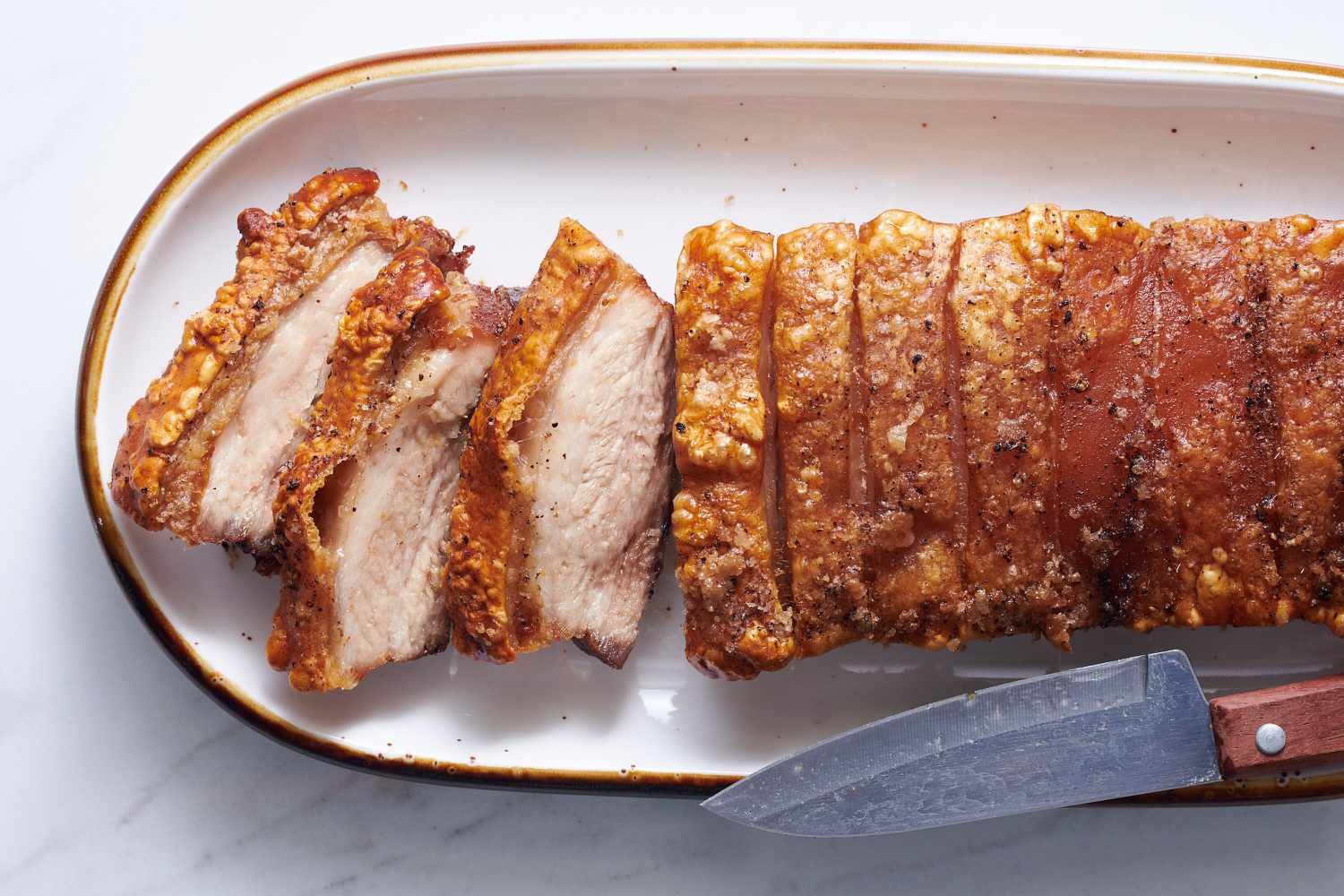This is an up-close photograph showcasing a meticulously prepared dish, featuring what appears to be either seasoned chicken or pork. The meat is encrusted in a vibrant orange breading and drizzled with a rich, red sauce. The dish is artfully sliced, with the first three slices arranged atop one another, revealing the succulent meat inside. The remaining slices are displayed with their tops up, concealing the meat from view. Presented on an elongated, oval-shaped plate, the dish is framed by a white surface adorned with black speckles and bordered by a brown rim. A knife, with a striking red cherry wooden handle and a short, gleaming silver blade, rests elegantly beside the dish.